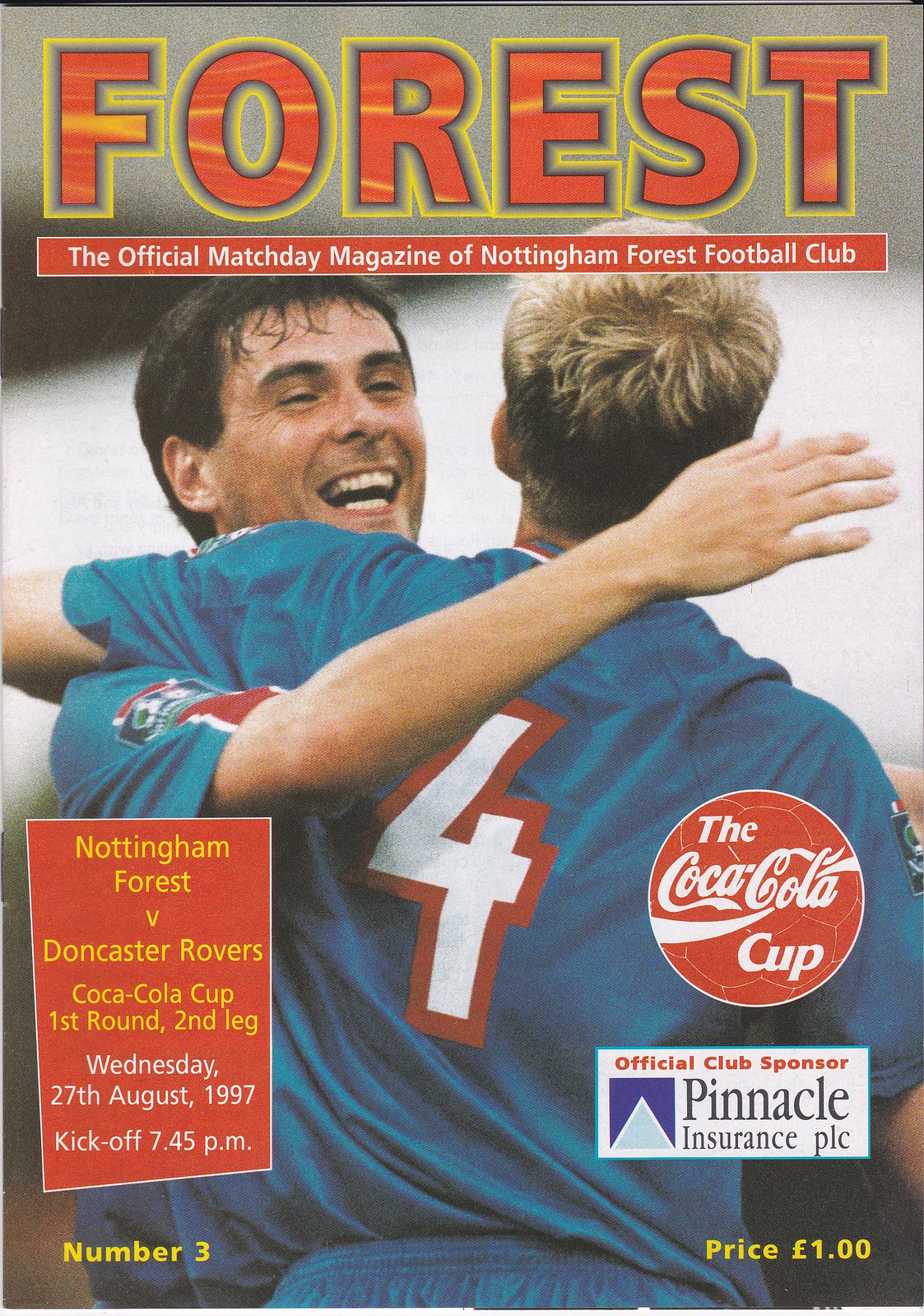This is the cover of the official match day magazine of Nottingham Forest Football Club. In bold red letters at the top, it reads "FOREST," with smaller white text underneath in a red text box stating, "The official match day magazine of Nottingham Forest Football Club." Dominating the center is a full-color photo of two soccer players, likely in their twenties, wearing blue uniforms. One player, seen from behind and wearing the number four, embraces the other, whose face is visible, smiling and sweaty with brown hair. They appear to be celebrating a moment on the field. In the bottom left, another red text box details the match: "Nottingham Forest V Doncaster Rovers Coca-Cola Cup first round, second leg, Wednesday, 27th August 1997, kickoff 7:45 p.m." The number three indicates the issue number of the magazine. On the right side, aligned vertically, are the Coca-Cola Cup logo and the note "official club sponsor Pinnacle Insurance PLC, price one pound."